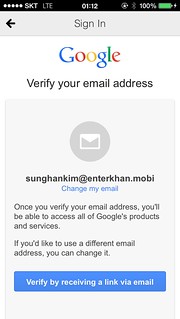Here is a detailed caption for the screenshot:

This is a screenshot of a Google verification screen captured on a smartphone. The indicators along the top reveal the smartphone's status: the device is connected via LTE as shown in the top left, the current time is displayed in military format as 01:12 (1:12 AM) in the center, and the battery is fully charged at 100% in the top right corner. 

The main content of the screen begins with a "Sign in" prompt at the top, followed by the Google logo. Below the logo, the text reads: "Verify your email address." In the middle of the screen, there is an icon resembling an envelope, surrounded by a grey circle. Directly underneath this icon, the email address "sunghangkim@entercon.mobi" is displayed, which appears to be the user's Google account email. Beneath the email address is a clickable option labeled "Change my email," allowing the user to substitute the current email address with a different one if needed. 

Further instructions on the screen explain that: "Once you verify your email address you'll be able to access all of Google's products and services. If you'd like to use a different email address you can change it." 

At the bottom of the screen, there's a prominent blue button with white text that says "Verify by receiving a link via email," which the user can click to proceed with verifying their email address.